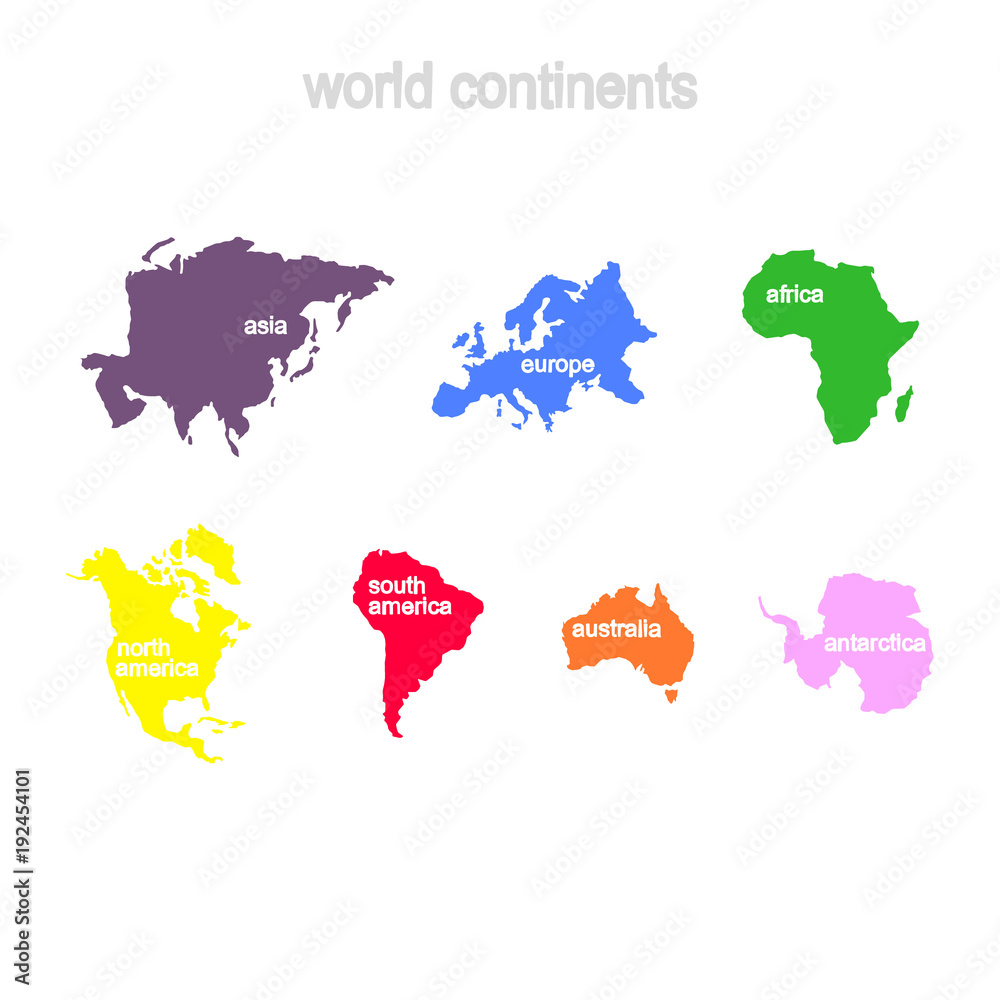This digitally created image features an all-white background with the seven continents outlined and labeled in distinct colors, presented in two rows. At the top of the image, "world continents" is written in light gray, all lowercase. The first row of continents includes Asia in purple on the left, Europe in blue in the center, and Africa in green on the right. The second row begins with North America in yellow on the left, followed by South America in red, then Australia in orange, and finally Antarctica in pink. Each continent is labeled within its outline in white text. In the lower left corner of the image, "Adobe stock number 192454101" is written vertically, with the text starting from the bottom and ascending. The continents are evenly spaced, with their relative sizes reflecting the actual proportions.